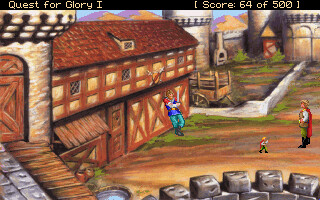This slightly rectangular, horizontally oriented image is a small screenshot from the video game "Quest for Glory I." A thin, black horizontal banner at the top displays yellow lettering, with "Quest for Glory I" on the left and "Score: 64 of 500" on the right. The main frame features a rustic country farmhouse that extends diagonally from the lower left corner toward the upper center. Leaning against this farmhouse with arms crossed is a character, adding a sense of daily life to the scene.

In front of the farmhouse, the ground is a combination of tan and blue hues, interspersed with patches of green grass. To the right side of the image, a person wearing a red cape stands facing the farmhouse, poised as if in mid-conversation. Adjacent to this person, slightly to the left, is a very small child, completing the image's evocative portrayal of a quiet, yet vibrant moment in the game.